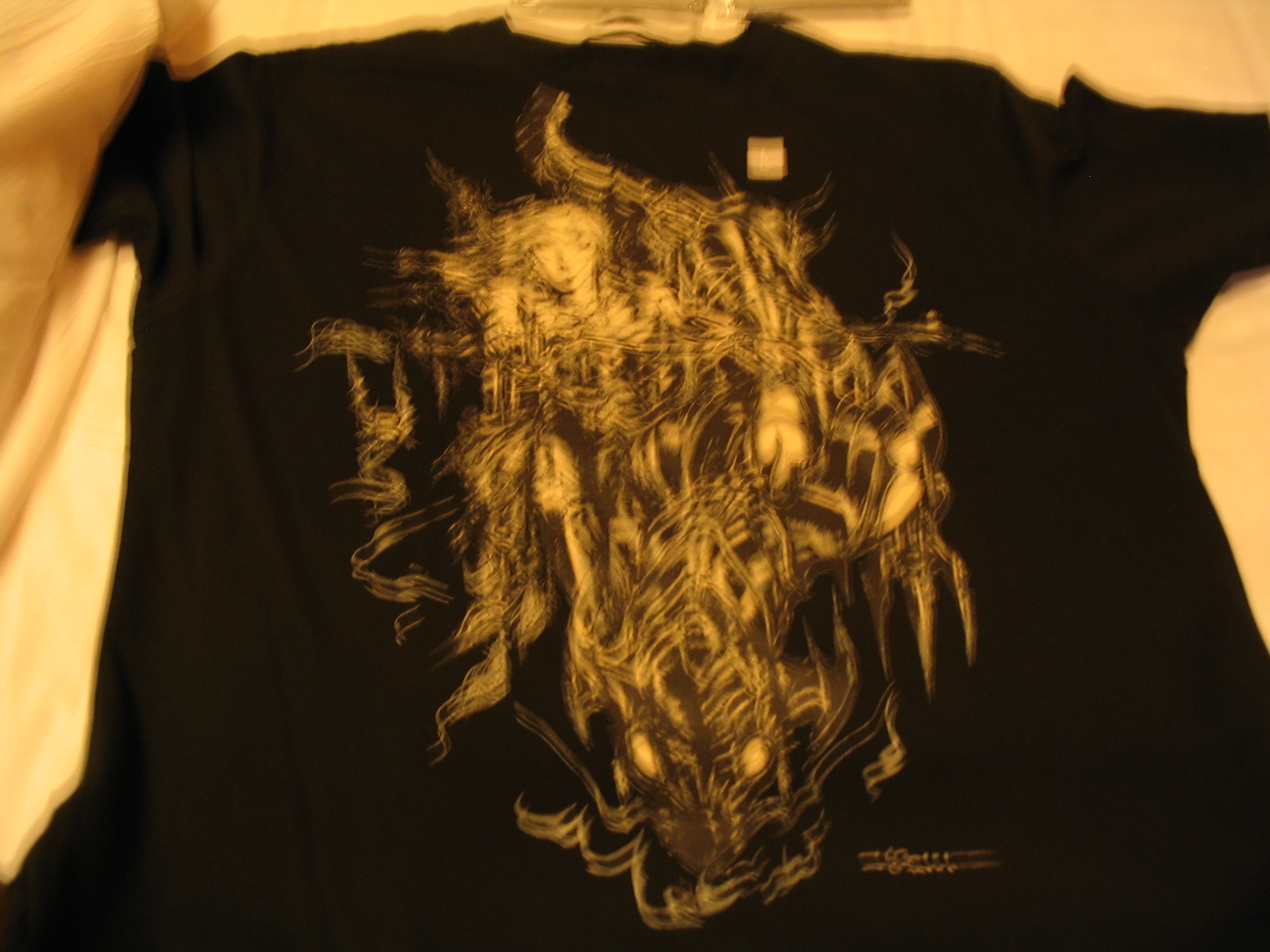A slightly blurry photograph captures a black t-shirt laying flat on what appears to be a white mattress. The shirt is hanging with a white hanger, which is visible through the collar. The front of the t-shirt features an intricate gold design. At the center of this design is the depiction of a woman, surrounded by elaborate gold wrappings that cascade across the front of the t-shirt. Near the bottom of the design, there's the subtle image of a creature's face, resembling a mouse, with distinctly gold eyes and nose.